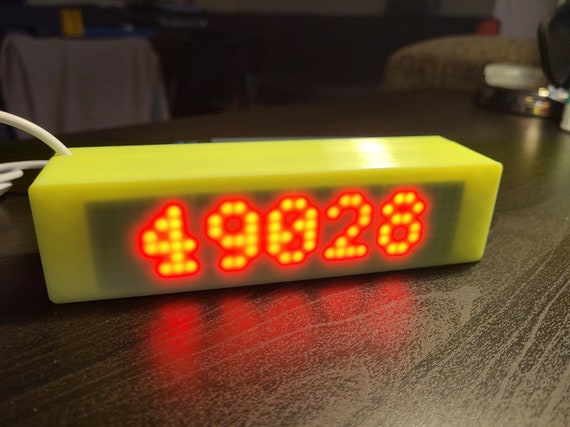The image showcases a bright yellow, rectangular plastic electronic device with a shiny surface, situated on a dark brown wood grain table, likely with a veneer finish. A thin white cord exits from the top left corner of the device, suggesting it is plugged in. Prominently displayed on the front of the device are LED numbers "49028," illuminated in bright red, each digit composed of small dots. A black circuit board is partially visible behind these numbers, enhancing the contrast against the bright display. The numbers' red glow subtly reflects off the shiny tabletop, adding a vibrant touch to the overall scene.